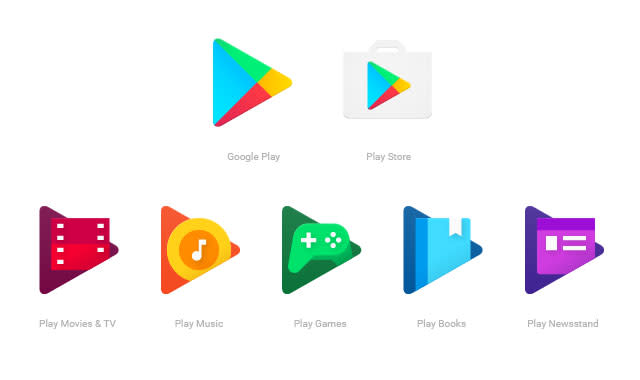This image displays seven Google app icons organized against a white background. At the top, there are two centered icons: the first is the Google Play Store icon, a colorful sideways triangle emblazoned in Google's signature hues of red, yellow, green, and blue, followed by the Play Store icon, a white briefcase adorned with the same multicolored triangle. Below them, five more icons form another row, each a right-facing triangle featuring distinct categories. From left to right, we see the red Play Movies and TV icon, featuring a filmstrip design; the orange Play Music icon with a white music note encased in a yellow circle; the green Play Games icon, showcasing a game controller; the blue Play Books icon, representing an open book; and finally, the purple Play Newsstand icon, symbolized by a newspaper. Each icon maintains a consistent triangular shape, and all are aligned horizontally, creating a visually cohesive arrangement.